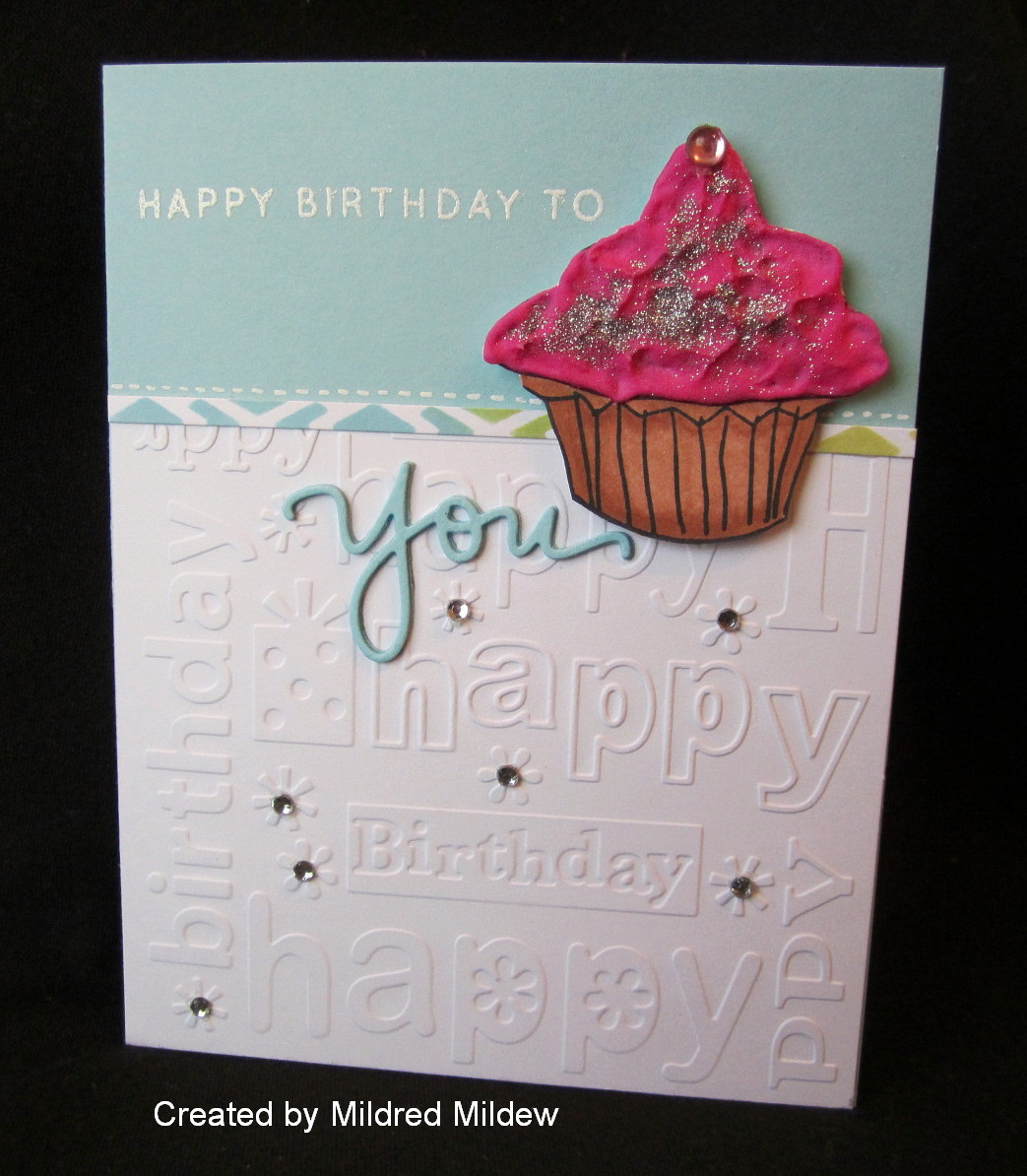This birthday card, created by Mildred Mildew, features an artistic design split into two distinct sections. The upper half of the card is a light turquoise color, adorned with the text "Happy Birthday to" in white, beside a beautifully detailed cupcake. The cupcake has pink frosting decorated with sprinkles and a jewel on top, with a brown base. Below the turquoise section, the majority of the card is white with intricate embossed and debossed textures, including raised white lettering that repeats the word "happy" multiple times. The word "you" appears in a cursive, light turquoise script towards the bottom of the card. Scattered throughout the white section are daisies embellished with metallic details and gems. Additionally, a horizontal strip with light blue and green lines runs across the card, adding a touch of color and pattern to the design.